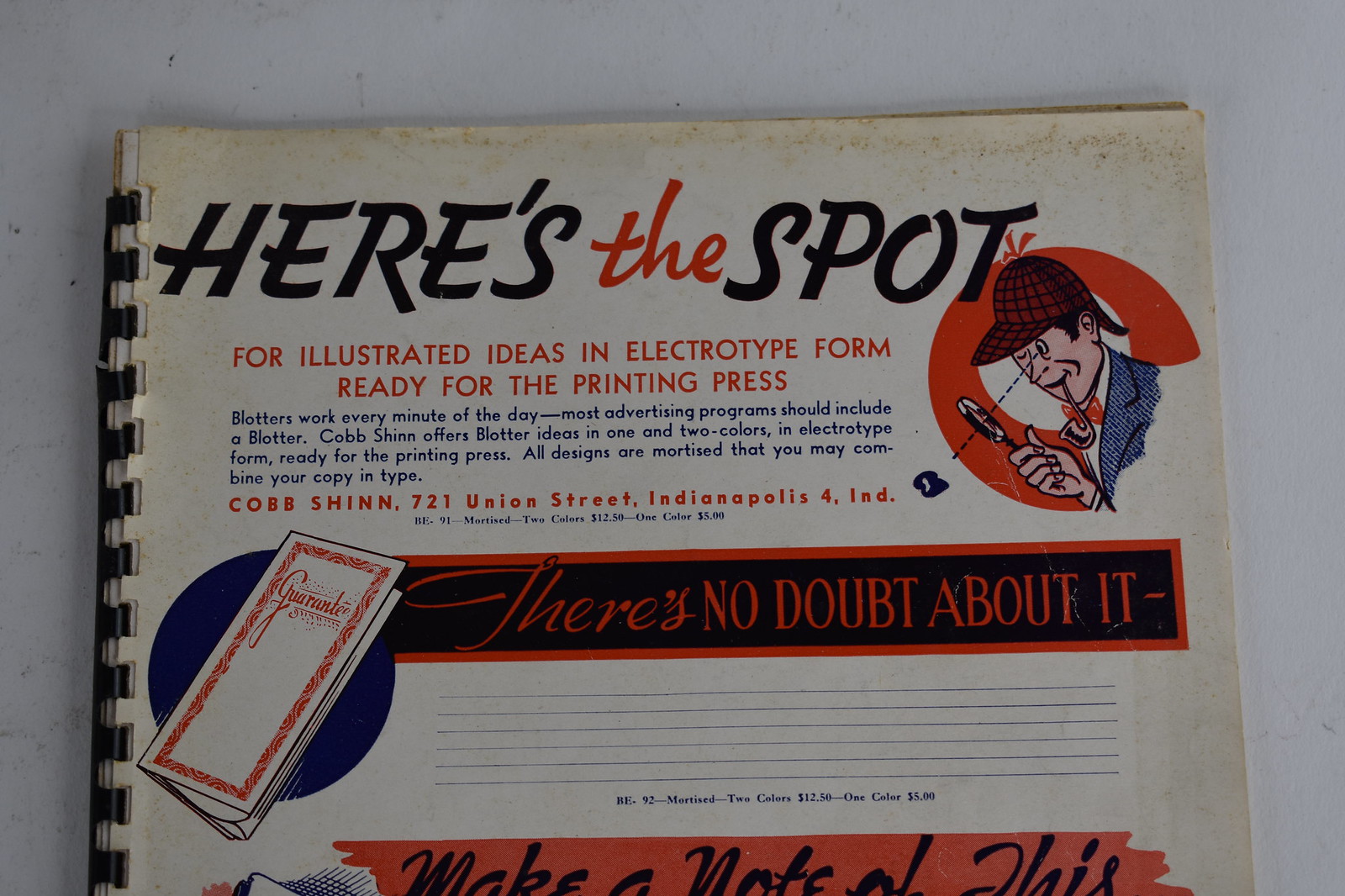The image displays a horizontal rectangular photograph of what appears to be an old manual resting on a dark gray surface. The manual is white with a black spiral binding along the left edge. Prominently, the title at the top reads "Here's" in large black letters, followed by "The" in red cursive, and finishing with "Spot" in large black letters again. To the lower right of the title, a small cartoon character resembling a detective is illustrated. The character, dressed in a blue coat, a red Sherlock Holmes-style hat, a white shirt, and a red bow tie, is depicted holding a magnifying glass with a red circle around him. Below the illustration, the text in large red letters reads, "for illustrated ideas in electro-type form, ready for the printing press." At the bottom of the cover, a black band with additional red text details further information, including the address "Cobb Shen, 721 Union Street, Indianapolis IV, Indiana," and phrases such as "Blotters work every minute of the day," emphasizing the value of blotters in advertising programs.